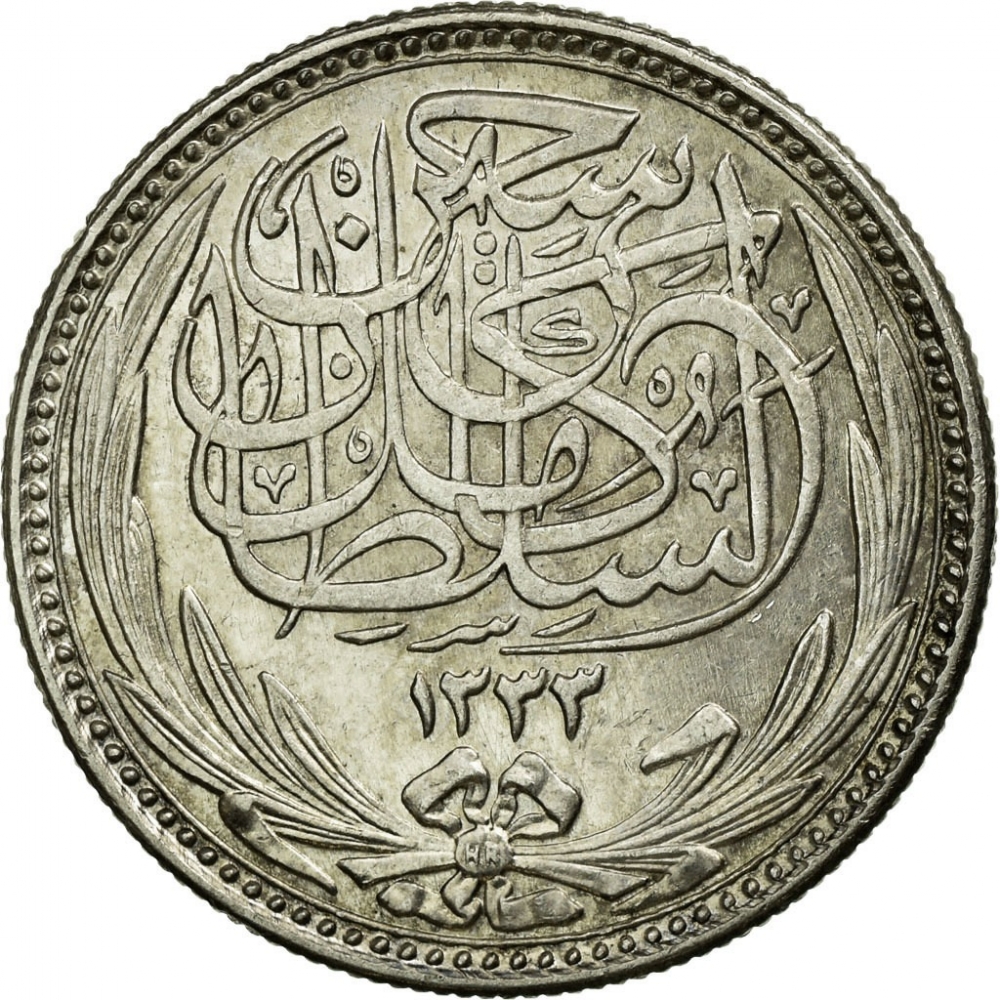This is a detailed zoomed-in image of a coin, showcasing intricate details and ornate designs. The coin features a silvery gray to light bronze color, with hints of darker silver and a slight greenish tint along the edges. The outer rim of the coin is adorned with small, evenly spaced circles. Within this rim, the main decorative elements include a bow at the bottom, tying together a pair of leaves or corn husks that rise up on either side. At the center of the bow, the initials "HR" can be seen. The coin's surface exhibits a script or calligraphy that is difficult to read, adding an element of mystery to its origin. The background of the image is plain white, drawing full attention to the coin's intricate and scuffed-up details.